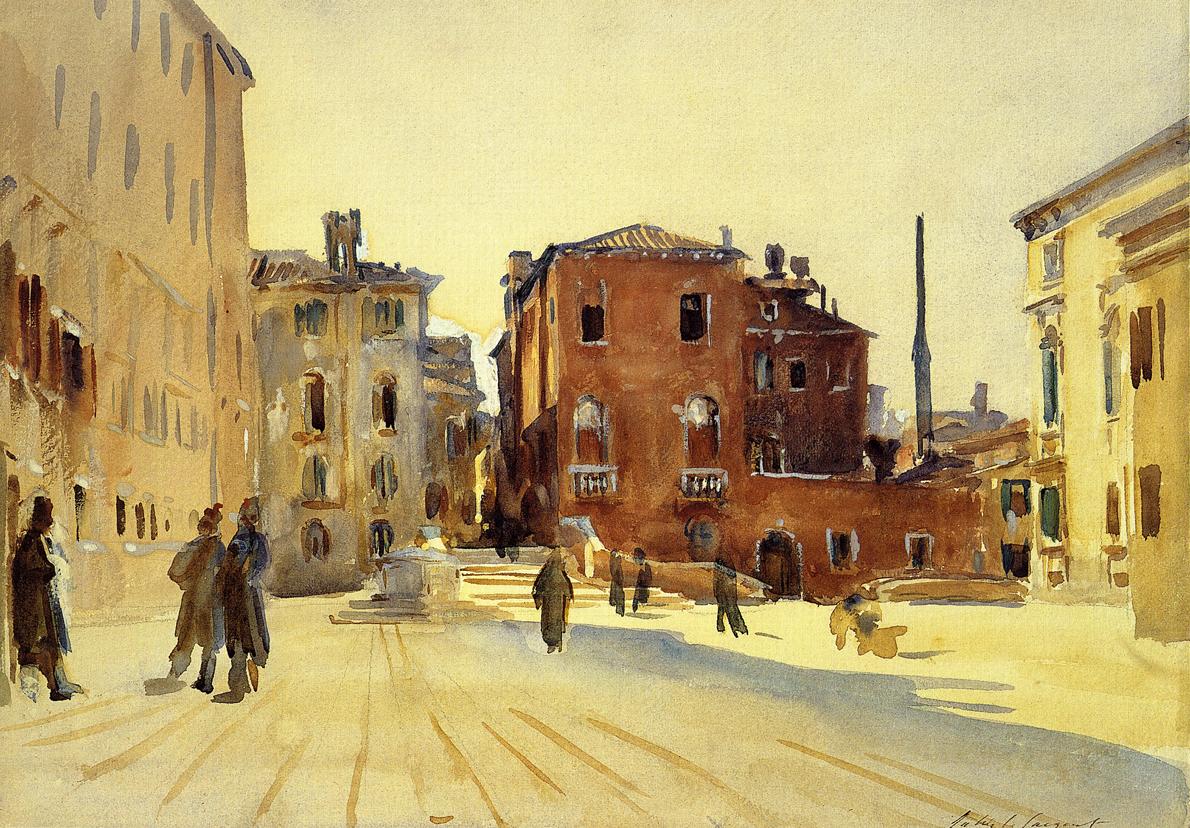This painting, devoid of any signature and seemingly from an era approximately 200 years ago, depicts a quaint small town or city street scene. Dominating the left-hand side is a large tan building adorned with numerous windows, in front of which three men, each donning hats and long coats, stand interacting. The man on the far left appears to be leaning against something, facing the other two. The middle ground reveals a smaller gray building adjacent to a striking red structure, behind which a bustling street can be seen. Here, several figures, their backs turned towards the viewer, are making their way along the street, with three or four visible at the foot of some stairs leading up and into an alley nestled between the buildings. The right side of the composition features a prominent brownish building with three floors, distinguished partly by a yellowish lower section and contrasting gray windows. Next to this, the edge of another bright yellow building emerges, its façade continuing beyond the frame. The street in the foreground is depicted in tan hues, interspersed with blue spots that may represent water or shadows. The entire scene is set against a plain white sky, lending a stark backdrop to the otherwise detailed urban tableau.